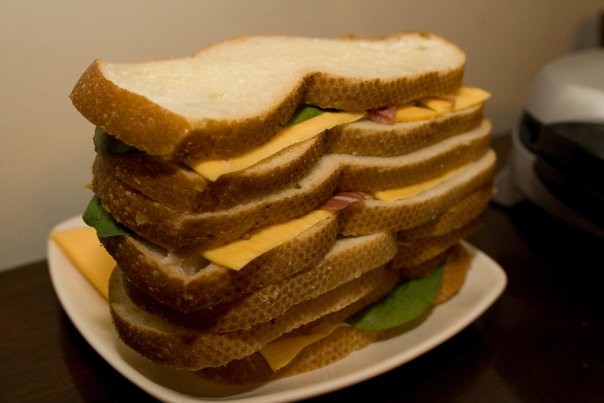This image showcases a multi-layered grilled cheese sandwich positioned on a white plate, which rests on a brown wooden countertop against an off-white wall. The sandwich is composed of seven slices of white bread with brown crusts, each layer containing yellow American cheese, green spinach, and assorted meats such as ham, prosciutto, and bacon. The vibrant layers of spinach peek out from between the slices, alongside the richly colored meats. Additional cheese pieces are scattered on the plate. To the right of the sandwich, a panini maker with a black and silver design can be seen, hinting at its role in preparing the towering sandwich. Multiple colors are evident in this image, including green, yellow, white, brown, silver, and black, adding to the visual richness of the depiction.